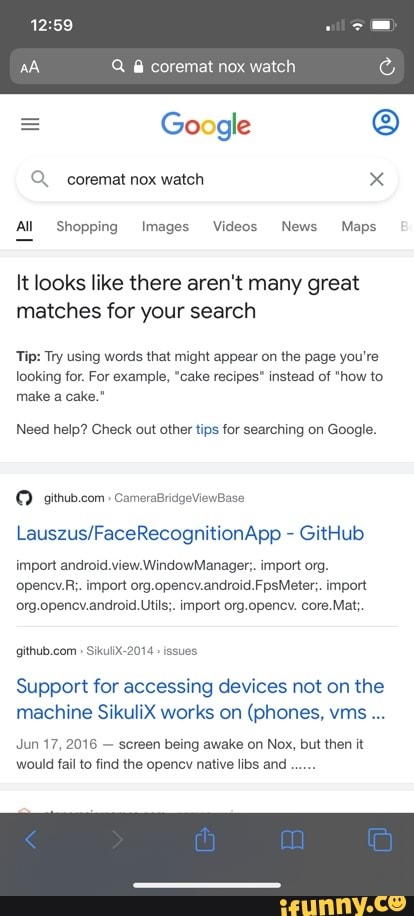This image is a screenshot of a Google search result page for "Cormat NoxWatch." The search results indicate that there are no relevant matches for the query, with a yellow-highlighted tip at the top advising users to try different search terms for better results. Beneath this suggestion, it offers general search tips, such as using specific keywords related to the topic of interest.

The first search result displayed is from GitHub, related to the "Lasus face recognition app," showing a snippet of technical information that includes the phrase "import Android View window manager," indicative of coding jargon.

The second result is also from GitHub, referencing support for accessing devices not on the machine, and mentions that "Sikulix works on phones VMS." Following this, there's a fragment about "screen being awake on Nox," with an incomplete phrase ending in "dot dot dot," hinting at a technical discussion.

In the bottom right corner of the screenshot, the watermark "iFunny.co" is visible in yellow, which is peculiar as iFunny is known for humorous content, yet this particular screenshot contains no apparent comedic elements.

Overall, the caption could be:

"A screenshot of a Google search result page for 'Cormat NoxWatch,' showing no relevant matches. The search tips recommend using more specific keywords. The first result from GitHub pertains to a face recognition app with technical details, while the second discusses device access and Sikulix compatibility. The iFunny.co watermark in the bottom right corner contrasts the lack of humor in the content."